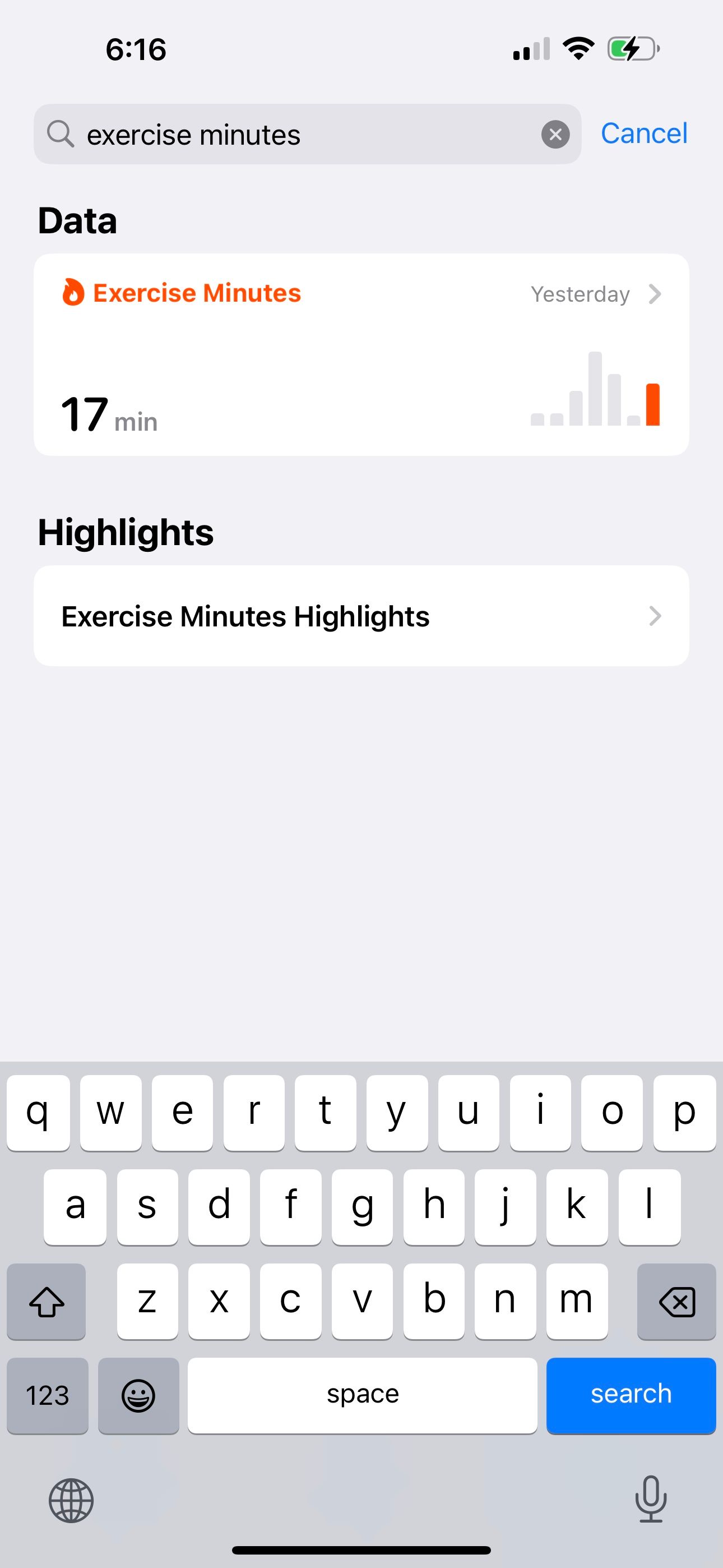The image depicts the screen of an iPhone displaying a health or fitness app. At the top left corner, the time is shown as 6:16, while the top right corner displays the network bars, Wi-Fi signal, and battery status. Just below, a search bar contains the text "exercise minutes," and a blue "Cancel" option is situated to the right of the search bar. The word "Data" appears next in black letters at the beginning of a white section.

In this white section, the term "Exercise Minutes" is highlighted in orange with a small fire symbol to its left. To the right, in small grey font, the word "Yesterday" and a right-pointing arrow are visible. Directly beneath "Exercise Minutes," the number "17" is prominently displayed in large black font, followed by the abbreviation "min" in smaller grey font. Beside these figures, a graph indicates the exercise minutes recorded across several days, with the current day's progress in orange showing approximately 50%.

Below the graph, the word "Highlights" is written in black letters, preceding another white section that includes the text "Exercise Minutes Highlights" and a grey arrow pointing to the right. The on-screen keyboard is visible at the bottom, indicating active text input.